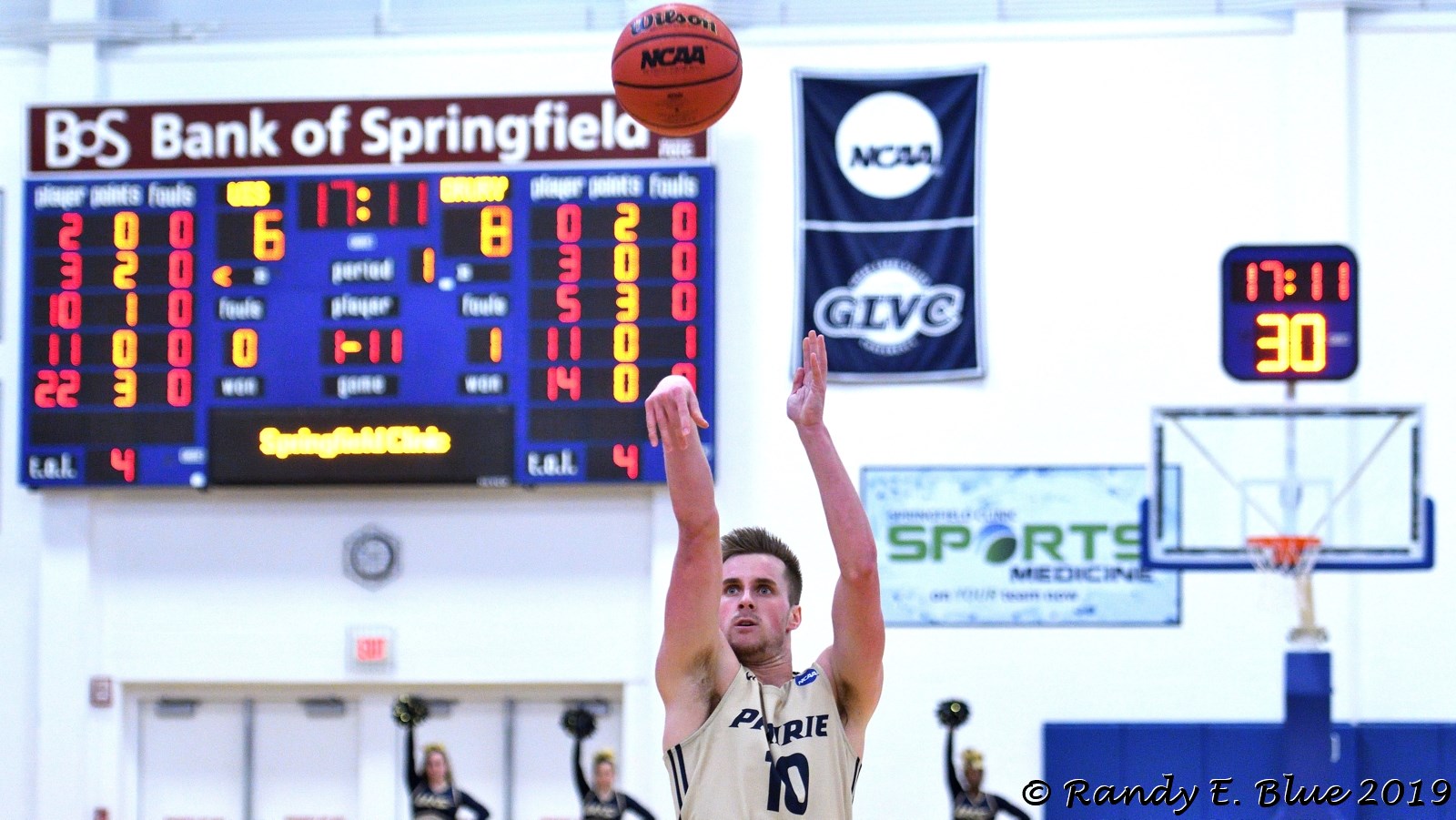In this detailed indoor gymnasium scene, we see a college basketball player, likely in his early 20s, executing a technically sound jump shot. The player, wearing a white sleeveless jersey with blue text reading "Prairie" and the number 10, has both arms poised perfectly—his right hand in a swan-like follow-through, and his left hand pointing skyward. The orange basketball, labeled with "Wilson" and "NCAA," is suspended in mid-air above him. In the background, several cheerleaders are visible, holding their pom-poms high in support. To the right, a digital scoreboard and shot clock are prominently displayed, with the clock showing "30" and "17:11". An all-blue scoreboard with LED lights indicates the game's details, underneath a rectangular sign for "BOS Bank of Springfield." Additionally, a navy blue cloth sign with "NCAA GLVC" is visible, highlighting the collegiate setting. There are double doors beneath an exit sign and another banner reading "Sports Medicine" completing the background details of the gymnasium.